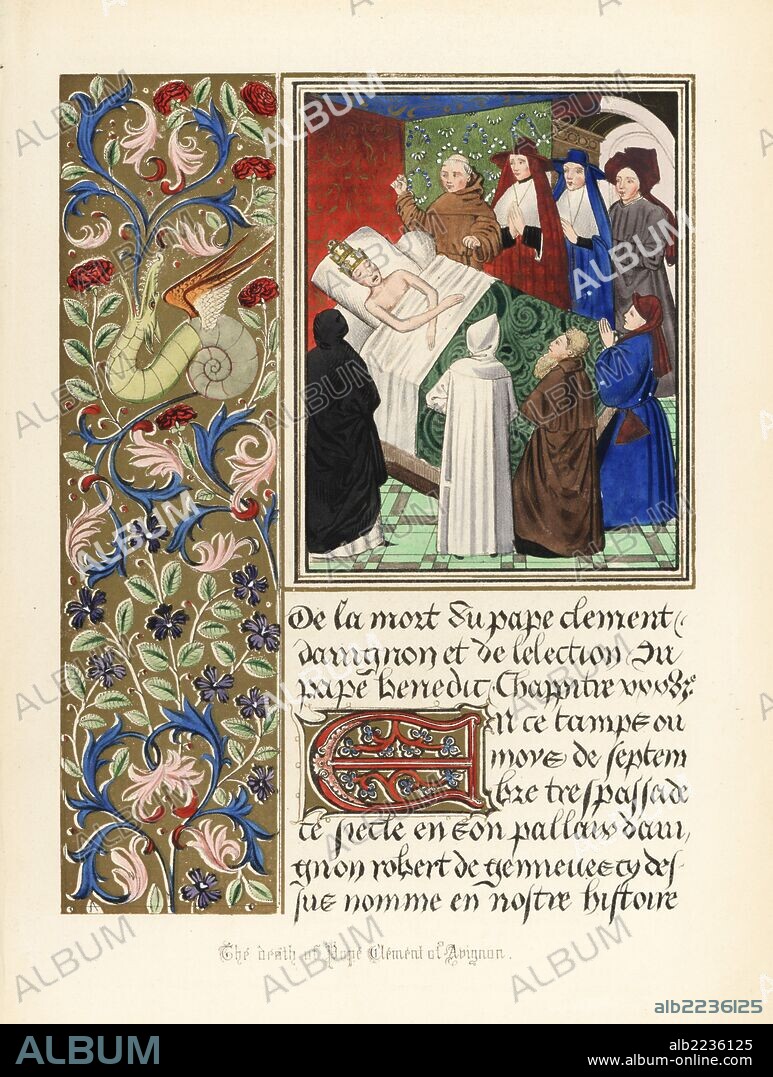This detailed illustration, perhaps from an old book, captures a historical scene laden with symbolic imagery. On the left side of the image, a vertical column embellished with intricate vines and flowers brings a touch of natural beauty. Adjacent to this, in the upper right section, lies a regal figure in a bed, draped in white covers and a distinguished green coverlet befitting royalty. Surrounding the bed are priests and attendants, their postures suggesting deep prayer or solemn observance. Close to the bedside is a menacing black figure, likely representing Death, adding an eerie presence to the scene. The room's walls are painted in a variety of colors: blue for the ceiling, red, green, and white arches possibly framing a door. The floor showcases a vibrant lime-green checkered pattern.

Below the image, black script, reminiscent of old-fashioned lettering, details the context of the scene. This writing may be in French, although it is not certain. Dominating the bottom section is a repeated word, "Album," which could imply a watermark or copyright notice. Finally, the inscription clearly identifies the subject of the depiction: "The Death of Pope Clement of Avignon." This caption provides a comprehensive and vivid description of the intricate and historical artwork.